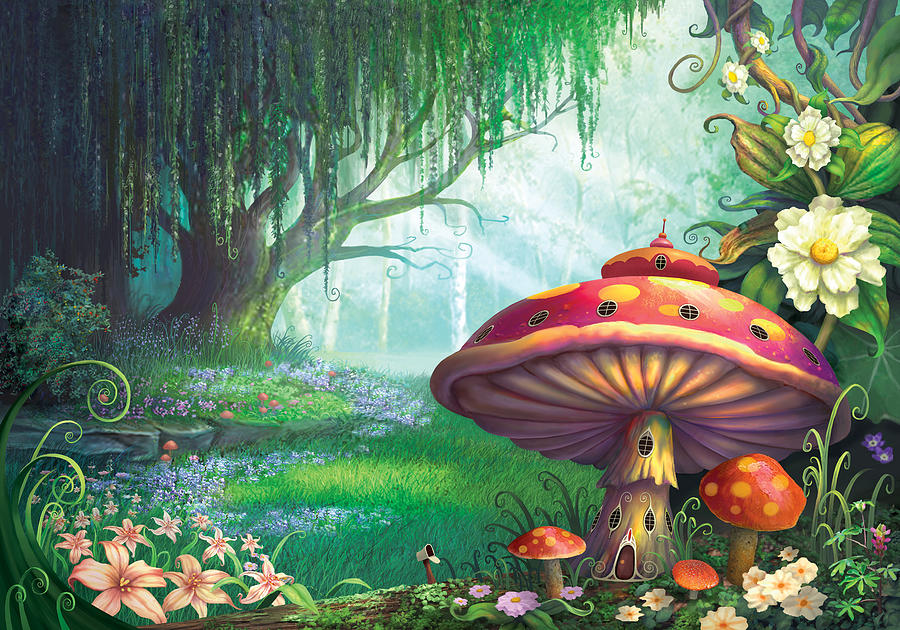This vibrant and detailed illustration depicts a fantastical outdoor scene, rich in whimsical elements. Dominating the left side is a grand tree with long, weeping leaves, reminiscent of a willow or oak, adding a sense of enchantment to the scene. The tree is surrounded by clusters of blue flowers, with pink five-petaled blossoms featuring yellow stamens in the left forefront, and delicately spiraled green fern fiddleheads adding lush greenery.

The right side of the image features a striking, large red mushroom house. Its stem has a charming face with open eyes and mouth, and it boasts a door and numerous windows, some with a widow’s peak, suggesting it’s a dwelling for magical creatures. Scattered below and around the main mushroom are smaller red mushrooms adorned with yellow spots, as well as orangish mushrooms with lighter orange dots. Adjacent to these mushrooms are clusters of white flowers, both with purely white petals and yellow centers and some with a yellow and orange middle.

Throughout the scene, various flowers in hues of pink, white, and purple dot the landscape. A subtle interplay of sunlight streaming through the center of the image adds a blueish light that enhances the fairytale-like quality of this fantastical forest.